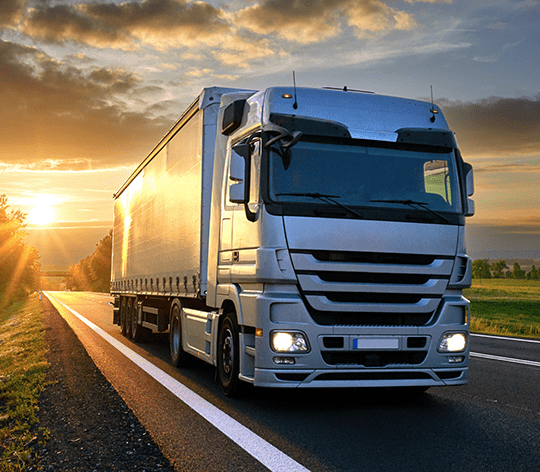The image showcases a modern, all-silver semi-truck with a bus-style front, featuring a clean, shiny appearance indicative of an AI-generated graphic. The semi-truck has a large windshield with dark tinted windows and prominent silver detailing, including a blank white and blue license plate. It is equipped with headlights that are on and orange lights at the top corners. The truck is hauling a silver cargo box and possesses multiple black wheels with potentially silver rims. The vehicle is situated on a black asphalt road marked by white solid lines on the outer edges and a dotted yellow line in the center, indicating a passing zone.

The landscape on either side of the road comprises expansive green grass, trees, and some black dirt. The sky overhead is a mix of blue and gray, dotted with tan-colored clouds that emit an orange hue due to the sun, positioned low on the left side of the image, suggesting it could be either setting or rising. Also in the distance, a bridge is faintly visible under the sun, adding depth to the scene. The picture exudes a serene, daytime ambiance with no other traffic present, enhancing its pristine, almost surreal quality.